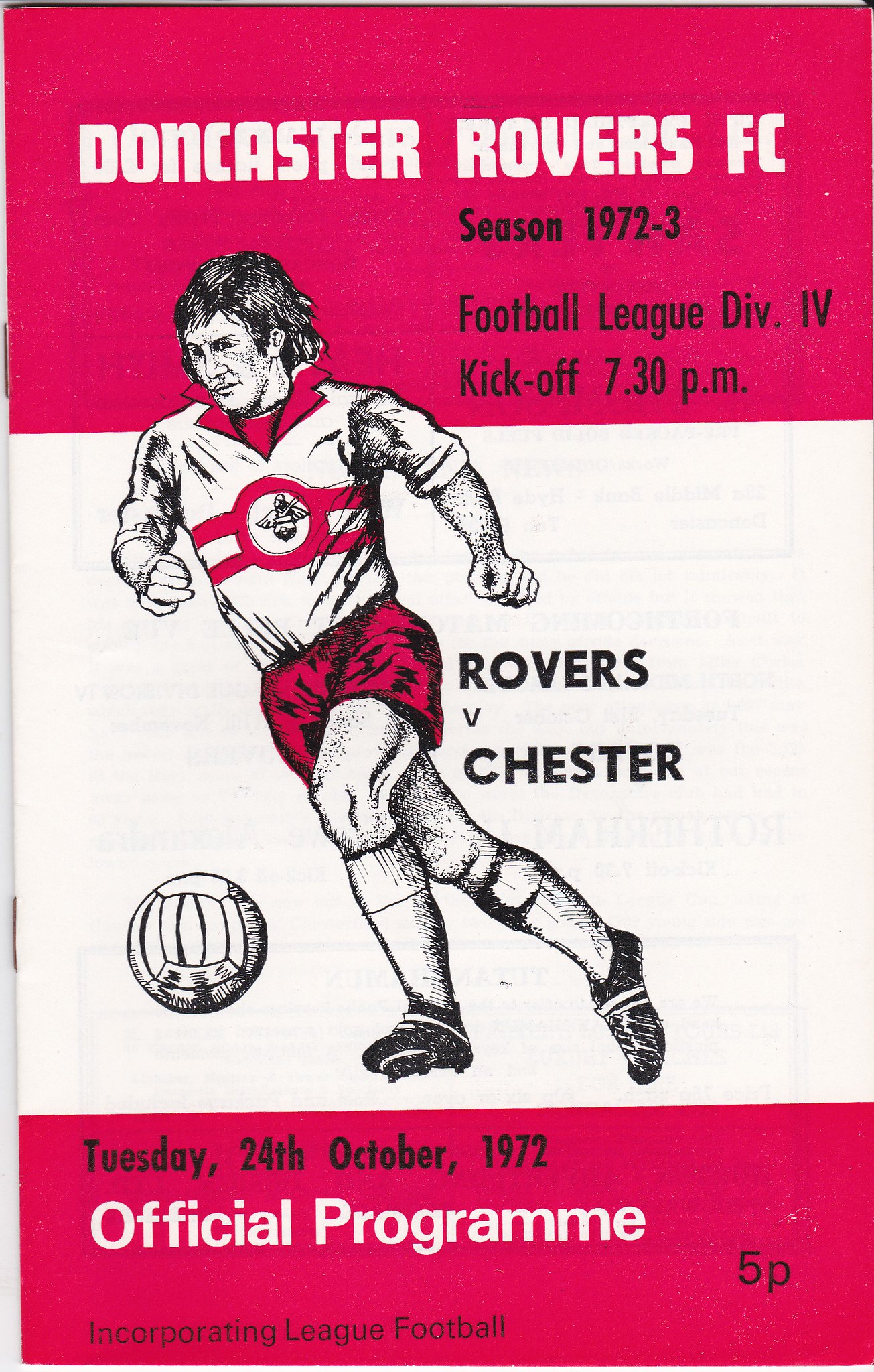This image depicts a vintage football (soccer) program cover from the 1972-1973 season, specifically for the match between Doncaster Rovers FC and Chester. Central to the design is a drawn image of a soccer player, wearing a red and white jersey with a red collar, red shorts, knee-high socks, and cleats, positioned slightly tilted to the left but centrally aligned. At his feet on the left is a white soccer ball. The background features a vibrant red, almost pink, and white color scheme, with white and black text. The top of the program reads "Doncaster Rovers FC Season 1972-3" in large white letters, followed by "Football League Division IV" in black. The kickoff time is listed as 7:30 PM. Further details include "Rovers vs. Chester" prominently displayed beside the player, and the date "Tuesday 24th October 1972." The bottom section of the cover turns red again with "Official Program Incorporating League Football" in white text, along with a price of "Five Pence."